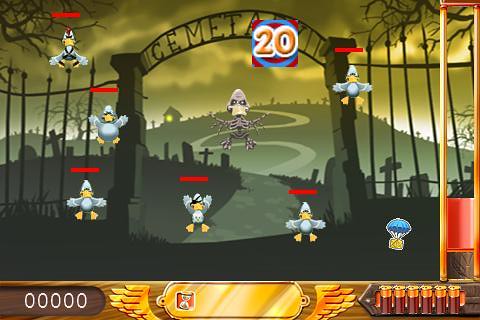The image appears to be a screenshot from a cartoony mobile game set in a gloomy cemetery at dusk or night. In the foreground, the cemetery gates are open, flanked by concrete or stone pillars topped with wrought iron spikes. The gate has an archway reading "Cemetery" in ornate metalwork, but part of it is obscured by a golden number 20, possibly indicating a bonus or score. A winding path stretches from the gates up through the hills in the background, passing by numerous tombstones and crosses silhouetted against a greeny-brown sky. A distant house with a single glowing green light in the window adds to the eerie atmosphere.

In the center of the image, a skeletal duck avatar stands out among six other ducks, which are adorned with various costumes. Each duck has a horizontal red health bar above its head, suggesting they are players' avatars. Suspended in mid-air are small boxes attached to parachutes, likely power-ups or collectibles. Along the bottom edge of the screen, several UI elements can be seen, including a sequence of zeros that may represent scores or stats, and a series of six shotgun bullet icons implying ammo count. There's also a bar, potentially indicating energy or power levels, and a small golden icon in the center which could denote a special status or achievement.